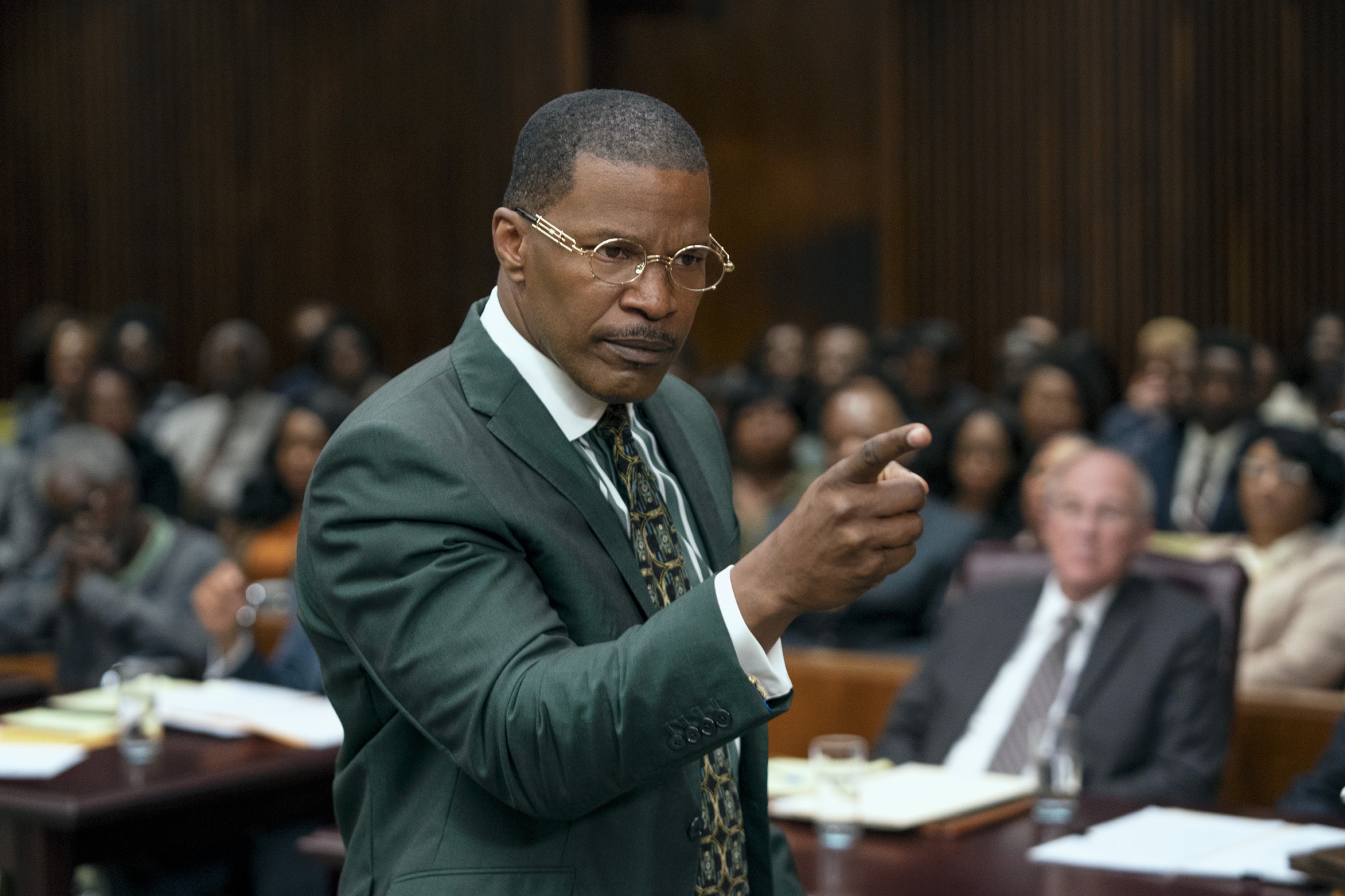In this detailed image, likely a still from a movie or TV show, Jamie Foxx portrays a lawyer in a courtroom setting. The courtroom is defined by brown wooden walls and an audience seated behind him, appearing blurry in the background. Jamie Foxx, a black man with short, neatly trimmed dark hair and a well-groomed mustache, commands attention as he points his right index finger assertively at someone off-frame. He wears gold-rimmed glasses, a suit in dark green hues, a green and white striped shirt, and a tie with green and gold accents. In front of him, there are two desks, each with water glasses and scattered papers, indicating an ongoing legal or governmental proceeding. The focus remains sharply on Jamie Foxx, capturing his intense expression and authoritative gesture.